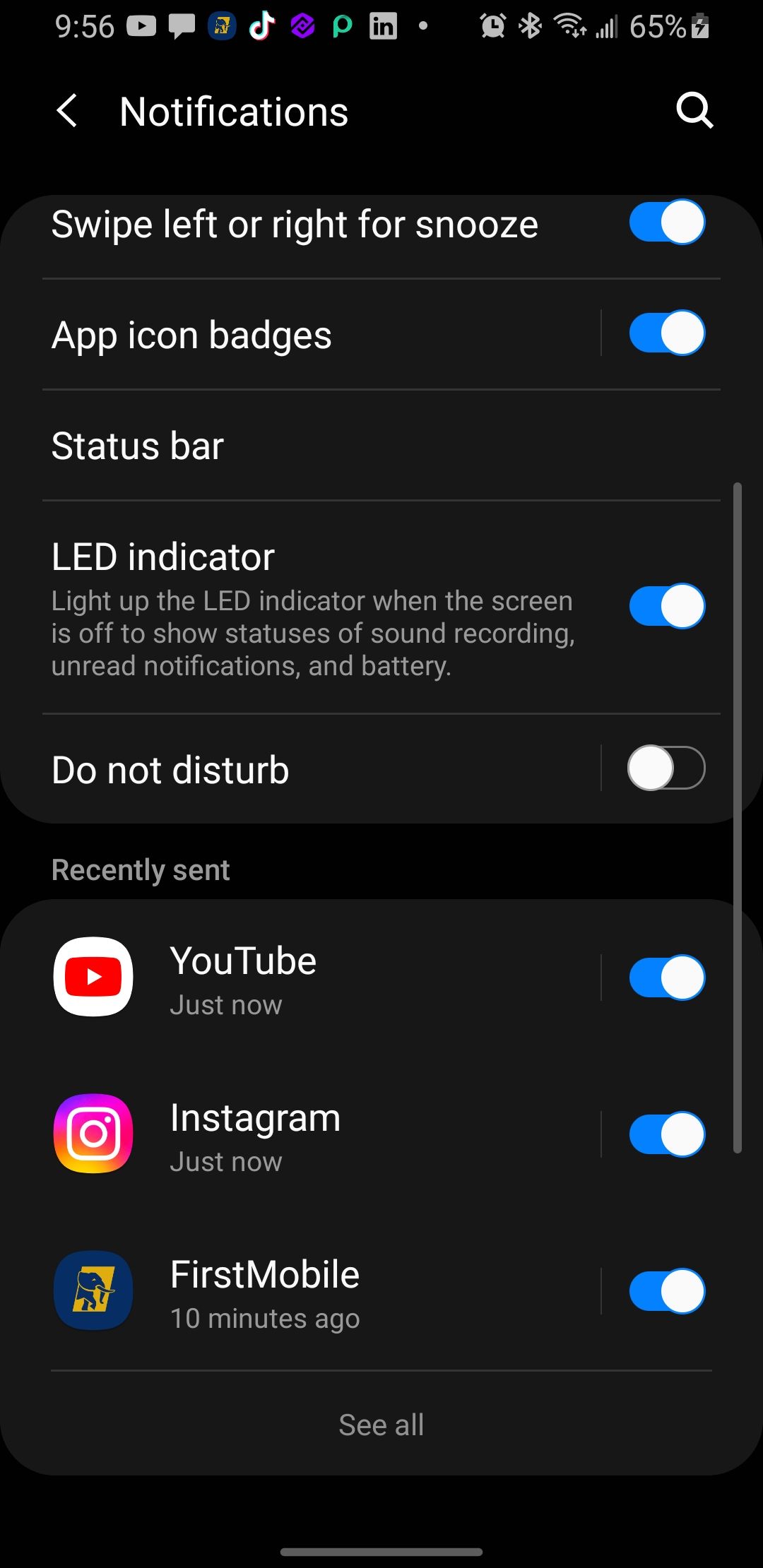This is a detailed screenshot of the notifications management settings on a non-Apple mobile device. The interface features white text against a dark background. The settings options are displayed in a sequential, top-to-bottom arrangement:

- **"Swipe Left or Right for Snooze"**: Enabled. This is indicated by the white switch positioned to the right.
- **"App Icon Badges"**: Enabled.
- **"Status Bar"**: Enabled.
- **"LED Indicator"**: This option is enabled. It indicates that the LED indicator on the screen will light up to show statuses, such as sound recording, unread notifications, and battery.
- **"Do Not Disturb"**: Not activated.

Additionally, the "Recently Sent" notifications section lists YouTube, Instagram, and First Mobile, all of which have notifications enabled. The layout and multiple icons at the top suggest that this is a screenshot taken from within the settings menu on an Android device.